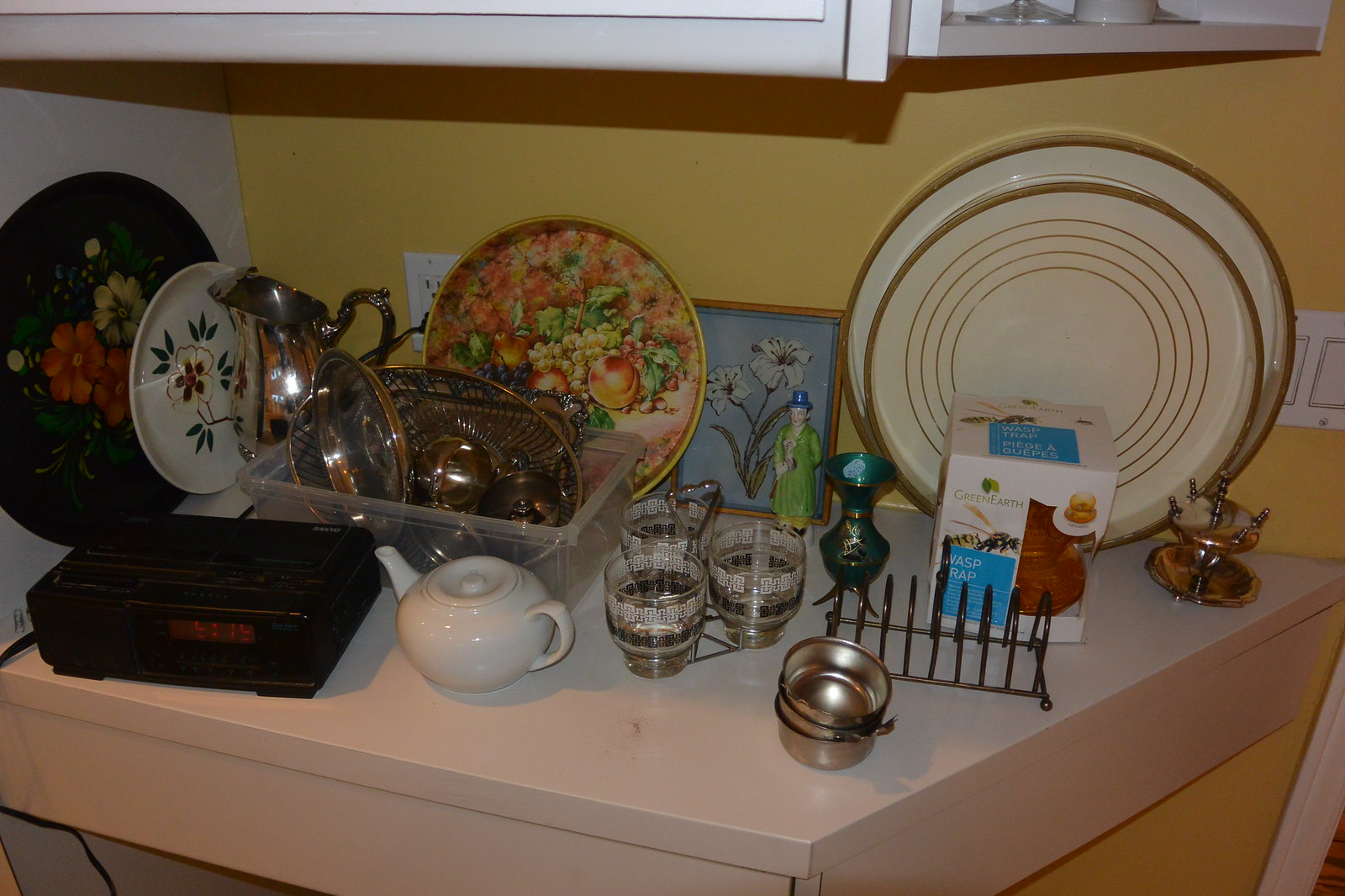In this detailed image, a small, rhombus-shaped countertop is presented, displaying a variety of items. The countertop, crafted from a reflective white material, is integrated into a wall painted a vibrant yellow. 

On the left side of the countertop, there is a round black plate adorned with intricate floral designs, propped up against the wall. In front of this, a similarly decorated white plate is positioned. Centrally placed on the countertop is a sleek black digital alarm clock. 

To the right of the alarm clock, a small white teapot sits, juxtaposed with a rectangular plastic bin filled with several silver objects, placed directly behind it. Leaning against the yellow wall behind these items is a plate featuring a colorful fruit design, slightly obscured by the outlet located in the top left corner of the plate. 

To the right of this fruit-themed plate, a square-framed drawing of a white flower hangs on the wall. Adjacent to this drawing, two white plates with elegant gold lines are displayed, completing the arrangement of objects on the countertop.